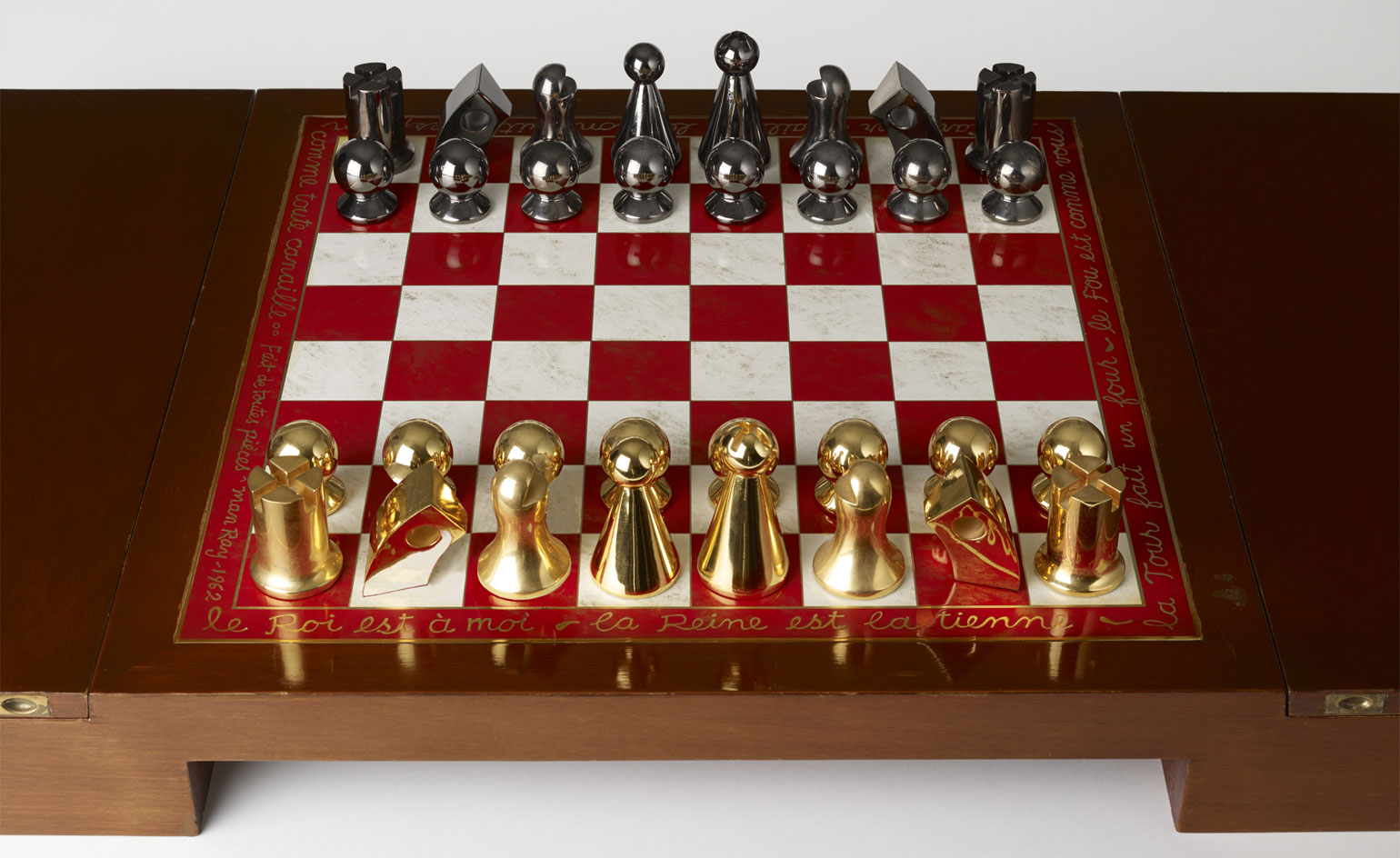This is a detailed photo of a chessboard set on a wooden game board table against a white backdrop. The tabletop and background wall are both white, enhancing the vibrancy of the chessboard itself, which is composed of alternating red and white squares. Surrounding the chessboard on a red background is an ornate, gold cursive script, likely in French, adding a sophisticated touch. At the back of the chessboard stand shiny silver chess pieces, while the front features equally polished gold pieces. The design of these pieces is unique, with the front pieces resembling small round balls on flat stands, and the back pieces varied in form—including tall structures topped with round balls and awkward rectangle shapes. The overall artwork of the board and pieces leans towards an abstract style, highlighting both elegance and distinctiveness in this luxurious chess set.